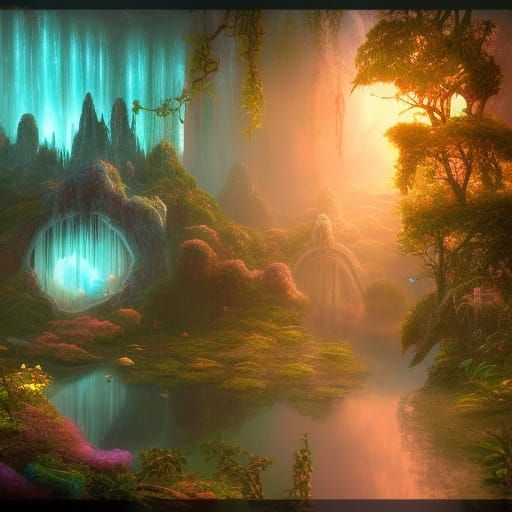In this mystical, fairytale-like scene, an artist's painting captures an ethereal forest bathed in a hazy glow. The upper part of the image features Spanish moss hanging from the trees, accompanied by vine-like structures, evoking an otherworldly ambiance. The scene is awash with greens, ambers, and bluish-green hues that play against each other to create a captivating light. On the right, unique, four-tiered trees and bushes frame the composition, while pools of water in the foreground reflect the enchanting surroundings.

In the center, an open, cavernous area emits green strands of light, adding a sense of depth and mystery. Further back, more strands of green light shimmer above the landscape. To the left, a small glimpse of a pink bush adds a splash of color amid the verdant scenery. The moss-covered hill in the background leads to an amber-colored light, suggesting a hidden realm or sanctuary, with sunlight casting an orangish glow to the right, enriching the fairytale atmosphere. Little islands adorned with purple flowers and lily pads dot the water surface, intensifying the scene's fantasy-film allure.